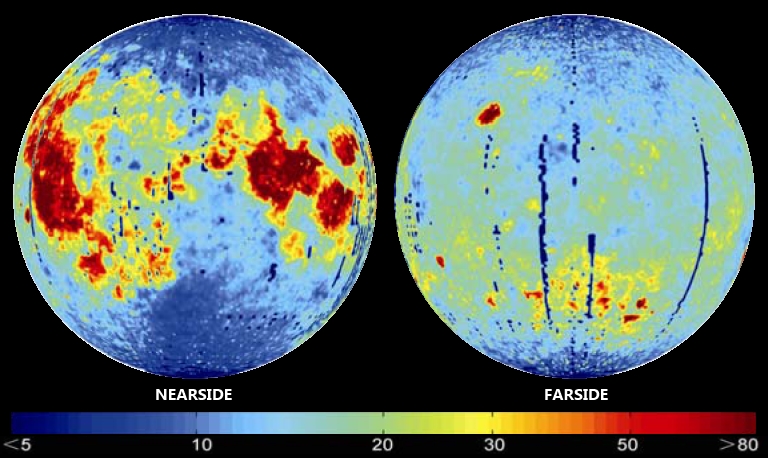The image features a black background with two distinct circles, each adorned with unique illustrations and labeled text. Both circles have a light blue backdrop, though their internal details differ significantly. 

The left circle, illustrating the concept of "nearsighted," features a more intricate array of illustrations. Prominent orange and yellow hues are visible on the left side of the circle, potentially symbolizing planetary or earthly elements bathed in vibrant, warm colors. Blue regions within this circle might represent water bodies.

In contrast, the right circle, labeled "foresight," is characterized by a simpler design. It predominantly showcases blue lines, with subtle hints of yellow and red, yet these colors are not as vivid as those in the left circle.

At the bottom of the image, a long, color-gradient strip transitions from blue to red, passing through yellow and orange tones. The strip is marked with numerical values starting from less than 5 and progressing through 10, 20, 30, and 50, up to 80, with a greater-than sign indicating the highest value.

This visually stimulating image employs color and symbolism to convey a comparison between nearsightedness and foresight, with a color gradient scale providing an additional layer of meaning.